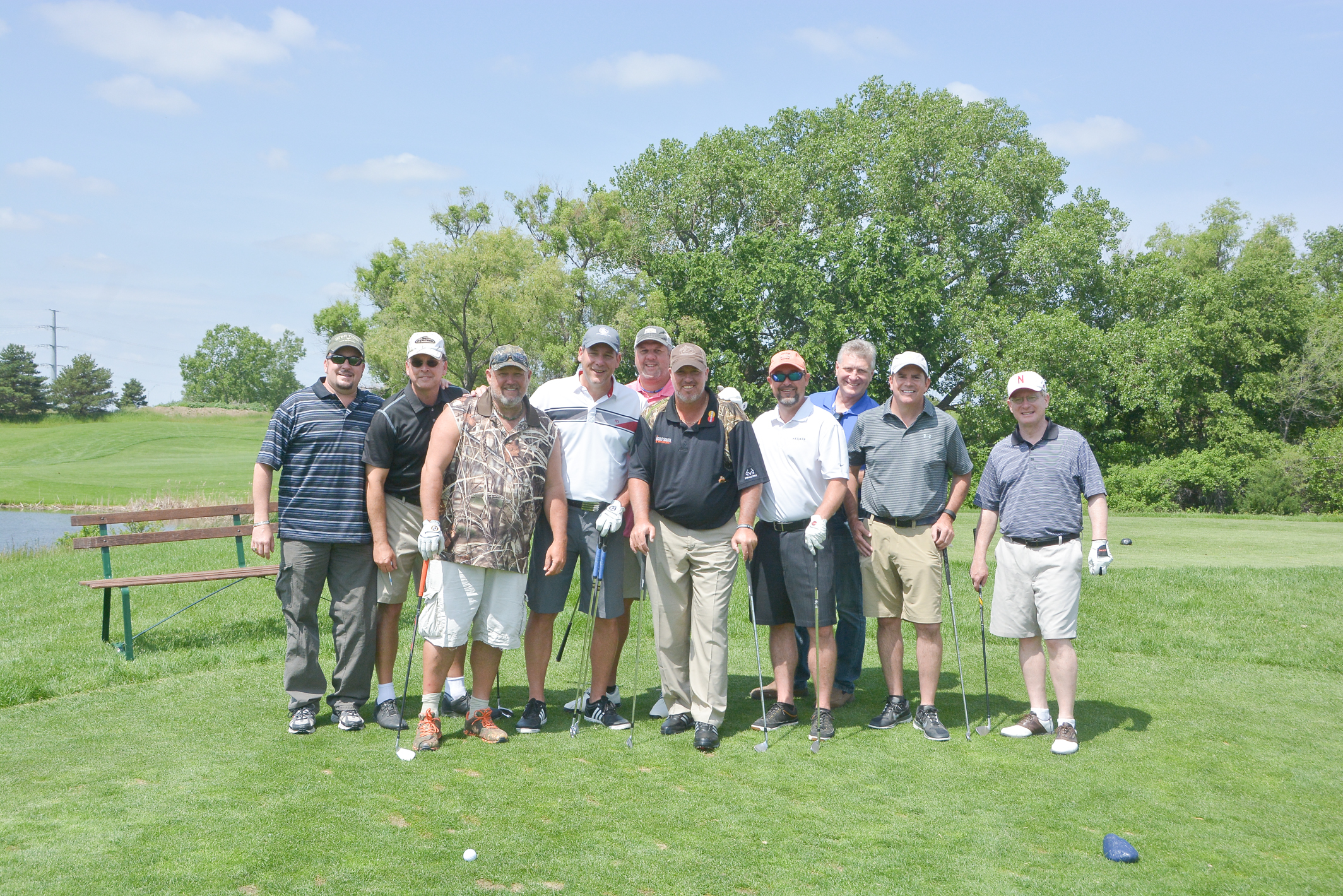This vibrant photograph captures a sunny day on a lush green golf course, showcasing a diverse group of ten men posing happily with broad smiles on their faces. Most of the men, positioned centrally in the image, are equipped with golf clubs and dressed in a mix of T-shirts, tank tops, and shorts suitable for golfing. Nearly all of them sport baseball caps, and four individuals are seen wearing sunglasses. In the lineup, there's a larger man in a blue shirt on the far left, alongside others in black, camouflage, white, pink, and gray attire, with some layering in the back.

The picturesque backdrop features a clear blue sky adorned with fluffy white clouds, and a dense arrangement of tall, leafy trees. A small pond glimmers on the left side of the scene, and a wooden bench sits slightly behind the group, enhancing the leisurely atmosphere. A golf ball is noticeably placed on the ground in the middle left of the image, underlining the sport-centric nature of the gathering. The combination of natural elements and cheerful camaraderie makes for a quintessential golf outing portrait.